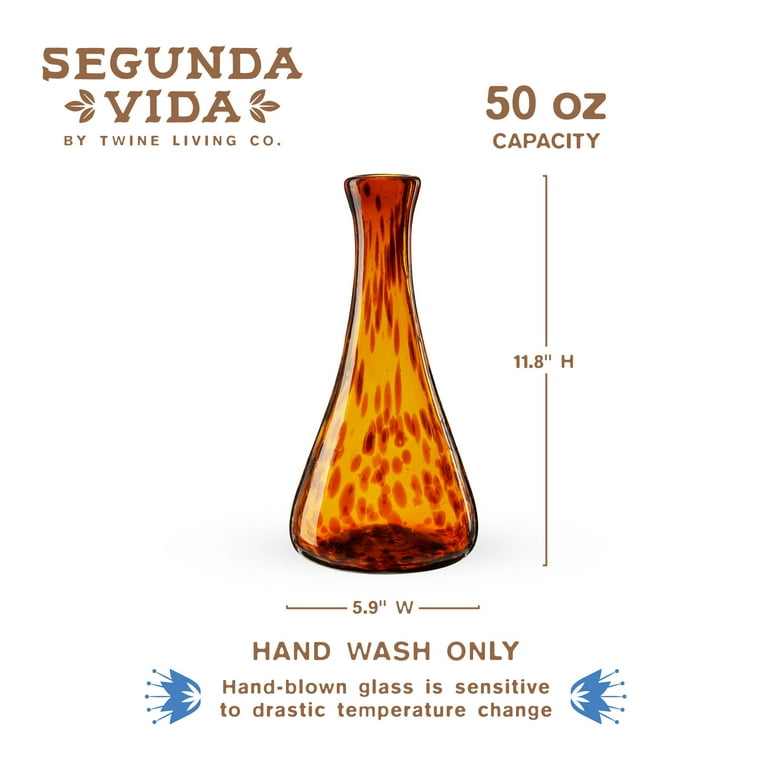This promotional image showcases a sleek hand-blown glass vase in shades of brown to orange. The vase, which fades from a darker brown at the top and bottom to a lighter, see-through brown in the middle, has a smooth and symmetrical design. It stands 11.8 inches tall with a base width of 5.9 inches, and has a capacity of 50 ounces.

In the top left corner of the image, the logo for "Secunda Vida" by Twine Living Company is displayed, featuring three leaves extending from either side of the word "Vida." To the right, "50-ounce capacity" is prominently written along with the dimensions of the vase. Below the vase, the instructions "hand wash only" are paired with a caution that "hand-blown glass is sensitive to drastic temperature changes." Additionally, there are icons resembling explosions flanking this warning, possibly indicating fragility due to temperature changes.

Set against a white background, the image effectively highlights the detailed craftsmanship and elegant form of the vase, emphasizing both its aesthetic appeal and practical considerations for its care.